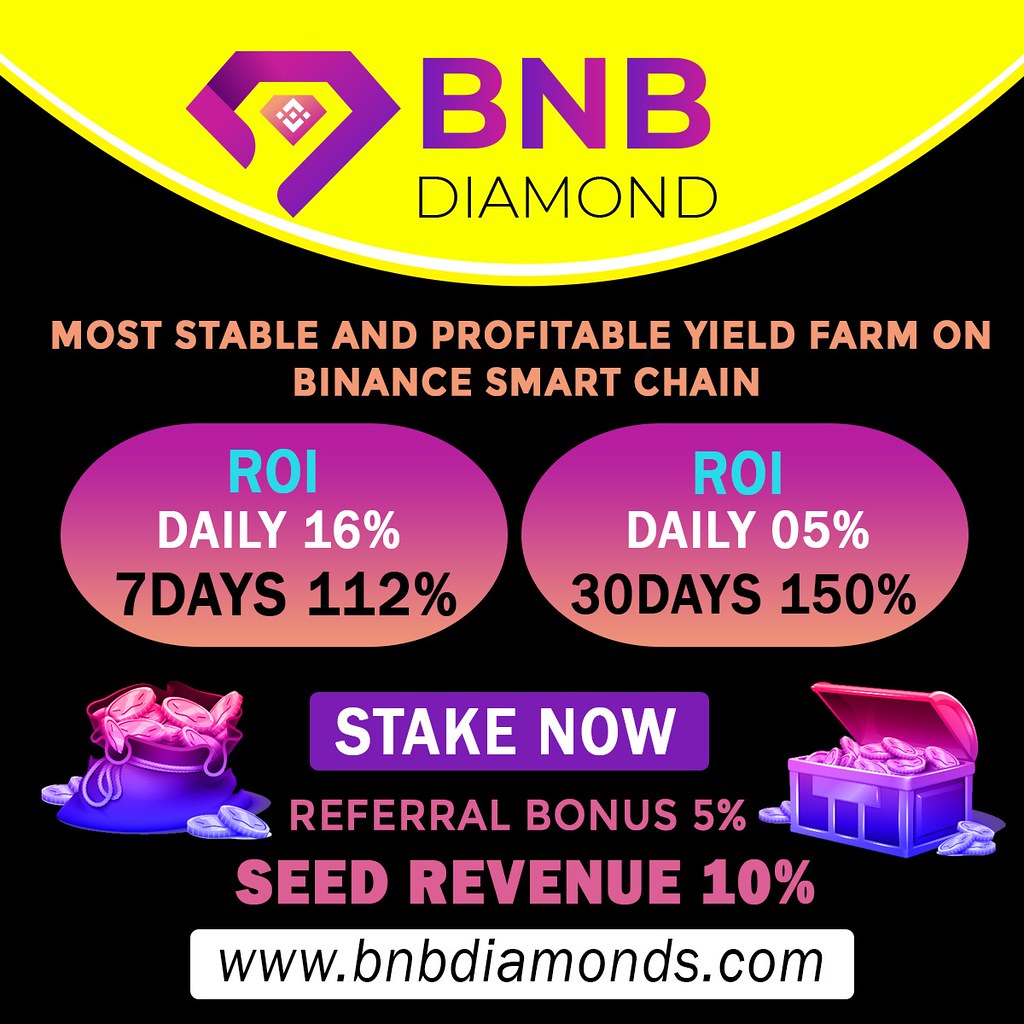This advertisement for BNB Diamond is set against a black background and highlights various colored graphical elements and text details. At the top, a white semicircle and a yellow semicircle prominently feature the BNB Diamond logo, which resembles a purple diamond with a pink diamond inside. Next to it, in white, are the words "BNB Diamond." Below this, in bright orange text, it reads "Most Stable and Profitable Yield Farm on Binance Smart Chain."

Further down, two purple ovals display return on investment (ROI) statistics: the left oval shows "ROI Daily 16%, 7 days 112%" while the right oval reads "ROI Daily 0.5%, 30 days 150%." In the center, a purple rectangle with the text "Stake Now" in white is flanked by graphical representations of a pile of gold coins and a treasure chest overflowing with coins.

Additional details include a purple section with the incentives "Referral Bonus 5%" and "Seed Revenue 10%." The bottom of the advertisement features a white box with black text displaying the website www.bnbdiamonds.com. The ad uses a vibrant mix of yellow, purple, white, orange, and black to draw attention to its key points.